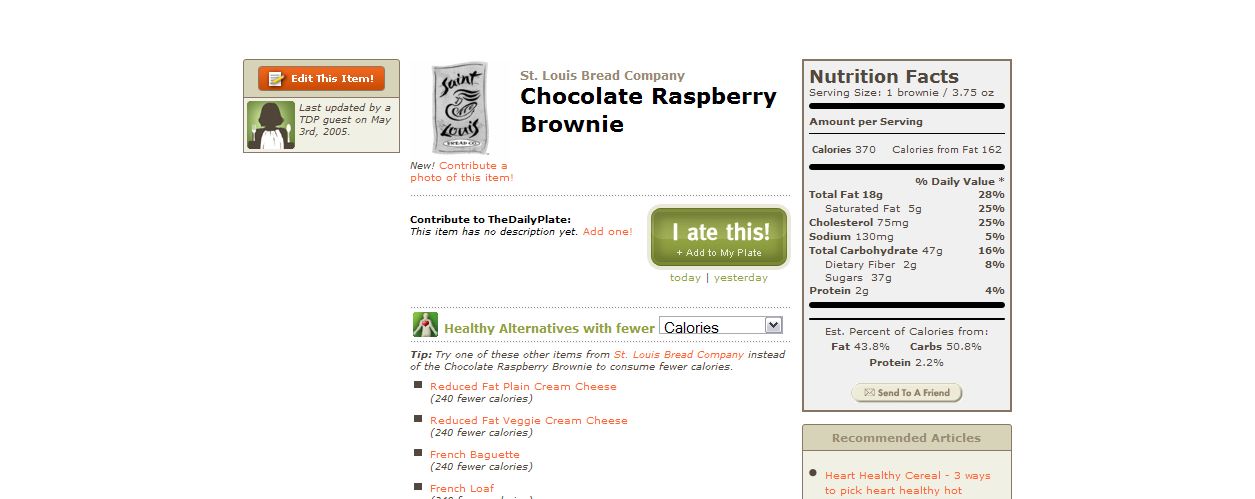This image appears to be a composite screenshot from an early 2000s era website, likely used for tracking calorie intake and nutritional information. The focal point of the webpage is a listing for a "Chocolate Raspberry Brownie" from the St. Louis Bread Company. In the top left corner, there is an orange box labeled "Edit this item," followed by another box stating, "Last updated by TDP guest on May 3rd, 2005." There's a small St. Louis logo next to these boxes, featuring a gray squiggly line. 

The main section of the page prominently displays the title "chocolate raspberry brownie" and a prompt encouraging users to "contribute to the daily plate." A green button labeled "I ate this, add to my plate" is available for users to log their food consumption. Below this, there's an option to look for "healthy alternatives with fewer" linked to a drop-down menu for various nutritional parameters.

To the right of the main content, a detailed nutrition facts box lists the calorie count as 370. Below this, there are different food items, potentially suggesting alternative choices, and a section for recommended articles that's partially cut off in the image. The entire background of this web page is white, adding to the basic and straightforward design typical of the era.